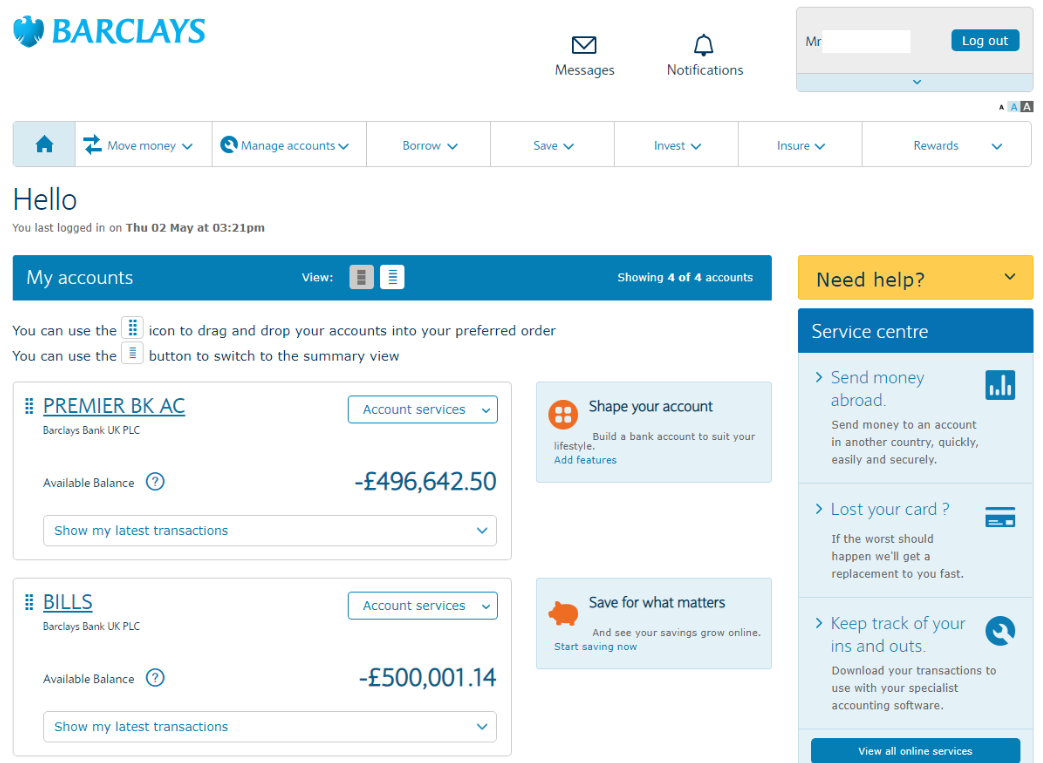This is a detailed screenshot of the Barclays Bank website, presenting a sleek and user-friendly interface. The background is predominantly white, with text primarily rendered in black. The website features a soothing color palette, including dusky blue and light blue blocks, with a notable yellow block labeled "Need Help."

In the top left corner is the iconic Barclays logo, depicting a blue eagle facing left, accompanied by the word "BARCLAYS" in blue, capital letters. To the right of the logo, the navigation bar includes an envelope icon for messages, a bell icon for notifications, and a grey block displaying "Mr." followed by a redacted name for privacy purposes. There is also an option to log out.

The primary navigation tabs include Home, More Money, Manage Accounts, Borrow, Save, Invest, Insure, and Rewards, each featuring a drop-down menu for further options. 

The Home screen welcomes the user with a message indicating their last login date and time: "Hello. You last logged in on Thursday, 2nd May at 03:21 PM." Below this, a large blue bar labeled "My Accounts" provides information about the user's accounts. These include a Premier Bank account and a Bills account, both showing significant negative balances.

To the right of the account information, there is an option titled "Shape Your Account," enclosed in a light blue rectangle. Below this section is a blue block with a small orange piggy bank icon and the message "Save for What Matters."

In the lower section of the screenshot, the yellow "Need Help" block stands out, followed by additional support options: Service Center, Send Money Abroad, Lost Your Card, and Keep Track of Your Ins and Outs, each accompanied by relevant symbols designed for easy navigation.